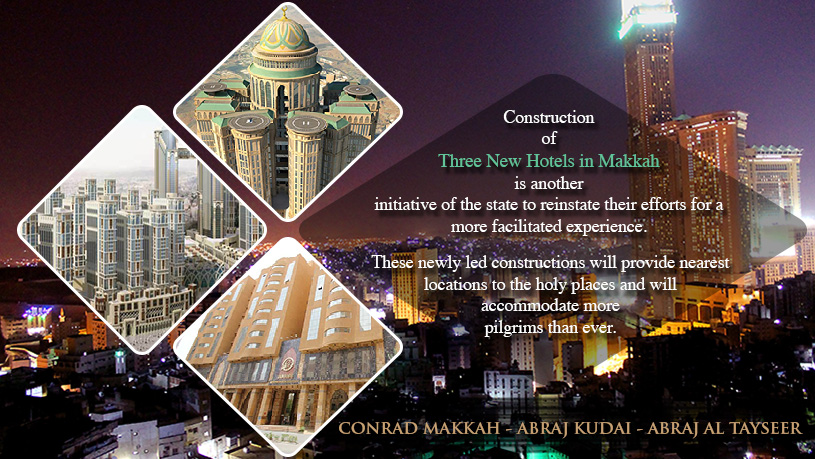The image portrays a modern cityscape at night, illuminated by the vibrant lights of skyscrapers in the background. Dominating the foreground are three diamond-shaped frames featuring images of new architectural constructions. The central frame highlights several cylindrical buildings that encircle a taller, domed cylindrical structure. To the left, another frame showcases a cluster of tall buildings, while the frame on the right reveals a twin building structure and a brown building. An overlaid text reads: "Construction of three new hotels in Makkah is another initiative of the state to reinstate the efforts for a more facilitated experience," emphasizing the state’s commitment to enhancing accommodations for pilgrims. The hotels—Conrad Makkah, Abraj Kudai, and Abraj Al-Taysir—are intentionally placed near holy sites to better serve pilgrims, indicating the construction's significance in Saudi Arabia for religious visits. The transparent section of the foreground text allows a clear view of the cityscape, seamlessly blending the information with the night scene.